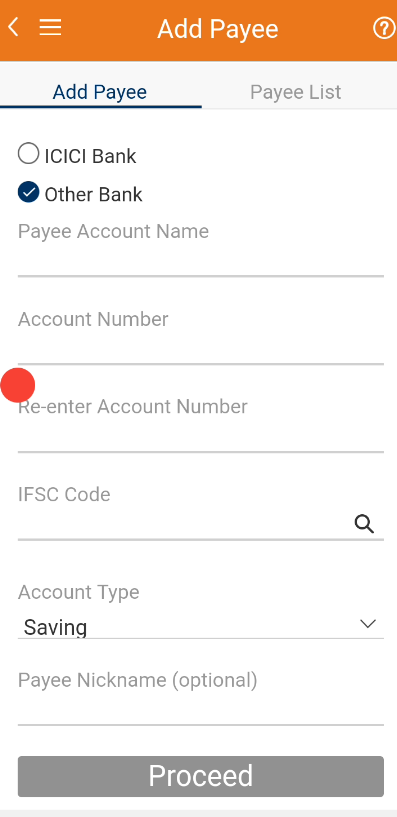The image depicts the user interface of a payment application. The top section features an orange bar with a white back arrow icon on the left, a three-bar menu icon next to it, and the title "Add Payee" centered in white text. To the right, there is a white question mark inside a circle.

Below the orange bar, a light gray bar divides the screen, which again shows the heading "Add Payee." On the left, the heading is in dark blue, underlined text, while on the right, a grayed-out option titled "Payee List" is visible, indicating it is not currently selected.

The main section beneath this starts with unordered and ordered payee options: 
- ICICI Bank (first circle, unchecked)
- Other Bank (second circle, checked)

Following this is a series of input fields:

1. Payee Account Name
2. Account Number
3. Re-enter Account Number
4. IFSC Code (accompanied by a magnifying glass icon to the right)
5. Account Type (pre-filled as "Savings")
6. Payee Nickname (optional)

Each input field is marked by a gray line below, awaiting user input. The only pre-filled data is "Account Type: Savings," which is the default selection for that field.